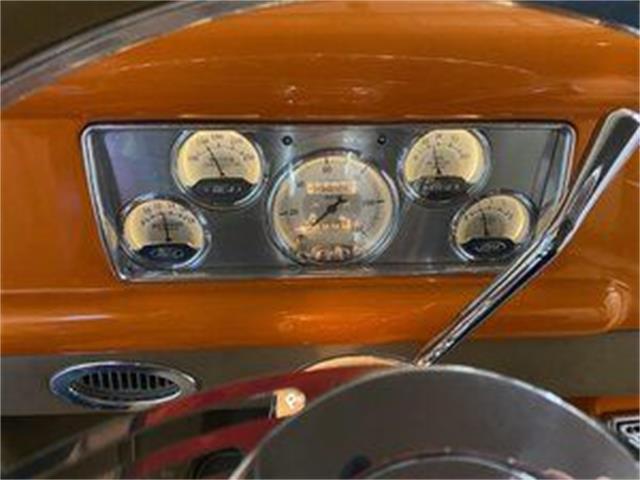The image portrays the dashboard of an old-fashioned car, reminiscent of models from the 1940s. The dashboard itself is primarily a rich brown wood with silver accents. Central to the dashboard is a silver inset panel featuring five circular dials, each with a slightly yellowish-tan background adorned with black numbers and lines. The middle dial stands out as the largest among them. The dials have black arrows for the markers and small black panels at the bottom of each. Flanking this arrangement, the top left and right corners are notably darker, possibly black or navy blue, adding depth to the design.

Below and to the left of this panel is a silver vent, while to the right, the gearshift selector, crafted in chrome, is positioned. The dashboard also includes additional chrome elements, such as a silver bar rising alongside the panel and a reflective chrome circle where the steering wheel would traditionally be found. At the bottom of the image, there is an oval cutout, also in silver, possibly another vent. The various chrome and silver details, along with the hints of red reflections, contribute to the vintage, mechanical allure of the dashboard.